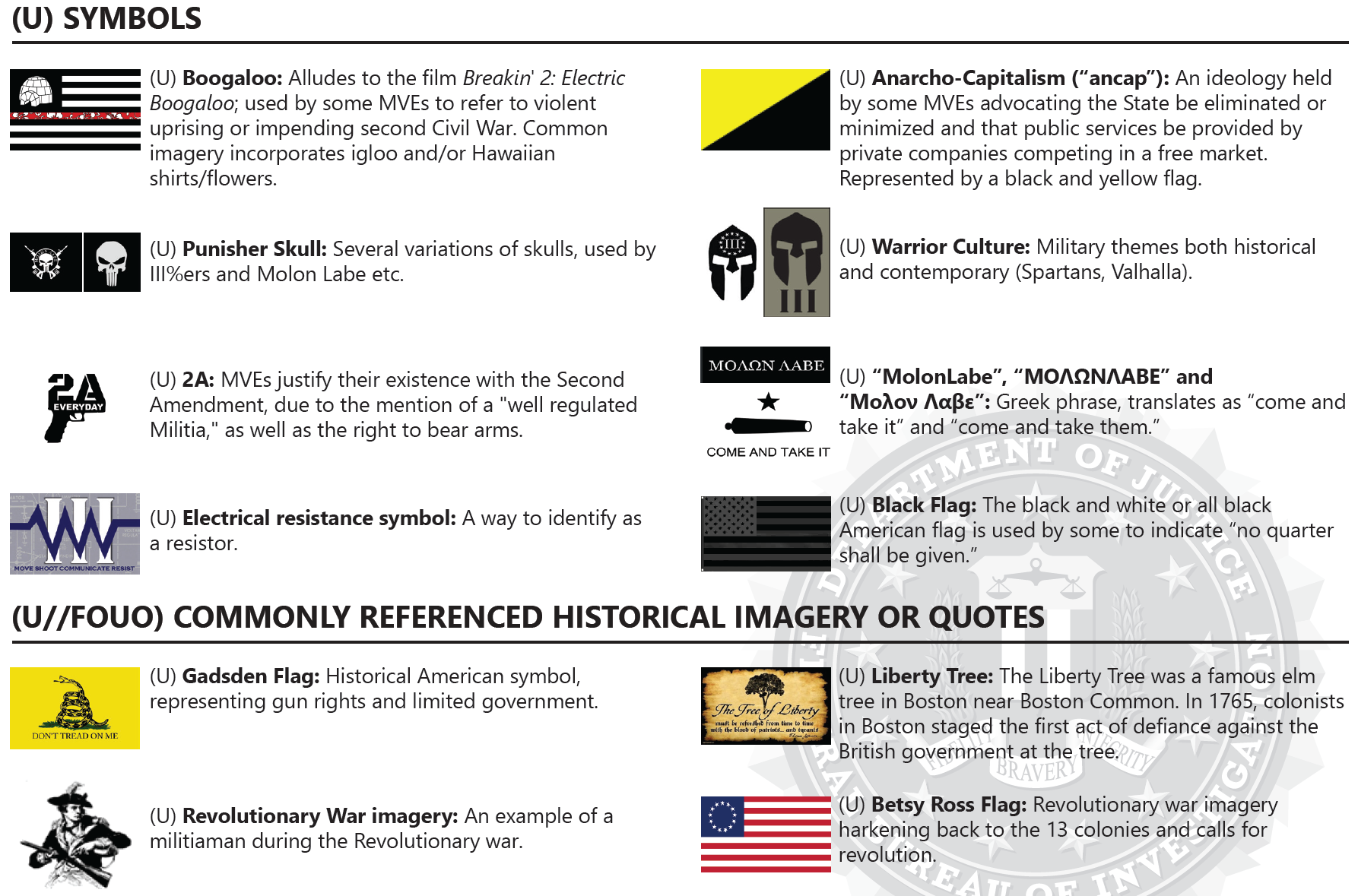The image is an educational infographic titled "(U) Symbols," divided into two sections. The first section features twelve symbols of various organizations, displayed in two rows of six symbols each. Each symbol is accompanied by a detailed description.

1. **Boogaloo Flag**: Resembling the American flag but with an igloo instead of stars, this symbol alludes to the film "Breaking 2: Electric Boogaloo." Used by some MVEs (Militant Violent Extremists) to signify a violent uprising or impending Second Civil War, it often incorporates imagery such as igloos or Hawaiian shirt flowers.
   
2. **Punisher Skull**: Variations of the skull are used by Molon Labe and Three Percenters, symbolizing defiance and self-defense.
   
3. **2A (Second Amendment)**: With a pistol illustration, this symbol justifies its existence with the Second Amendment's mention of a well-regulated militia and the right to bear arms.

4. **Electrical Resistance Symbol (Ω)**: A resistor symbol identifying resistance in electrical contexts.

5. **Anarcho-Capitalism Flag**: Represented by yellow and black triangles, this flag signifies an ideology held by some MVEs advocating for minimal or no state intervention and public services provided by private companies in a competitive free market.

6. **Warrior Culture Helmet**: Depictions of military themes, historical and contemporary, including Spartans, Valhalla, and the Greek phrase "Molon Labe" (Come and Take It).

7. **Black Flag**: An all-black or black and dark gray American flag indicating no quarter shall be given.

The second section, titled "Commonly Referenced Historical Imagery or Quotes," features four more symbols:

8. **Gadsden Flag**: A yellow flag with a coiled snake, symbolizing American independence and limited government.
   
9. **Revolutionary War Imagery**: An illustration of a militiaman from the Revolutionary War.
   
10. **Liberty Tree**: Iconography of the famous Boston elm tree, a site of early American resistance against British rule.
   
11. **Betsy Ross Flag**: An early American flag representing the original 13 colonies and evoking Revolutionary War sentiments and calls for revolution.

The color palette includes black, yellow, white, red, blue, and gray tones, providing a visually muted yet symbolically rich presentation.